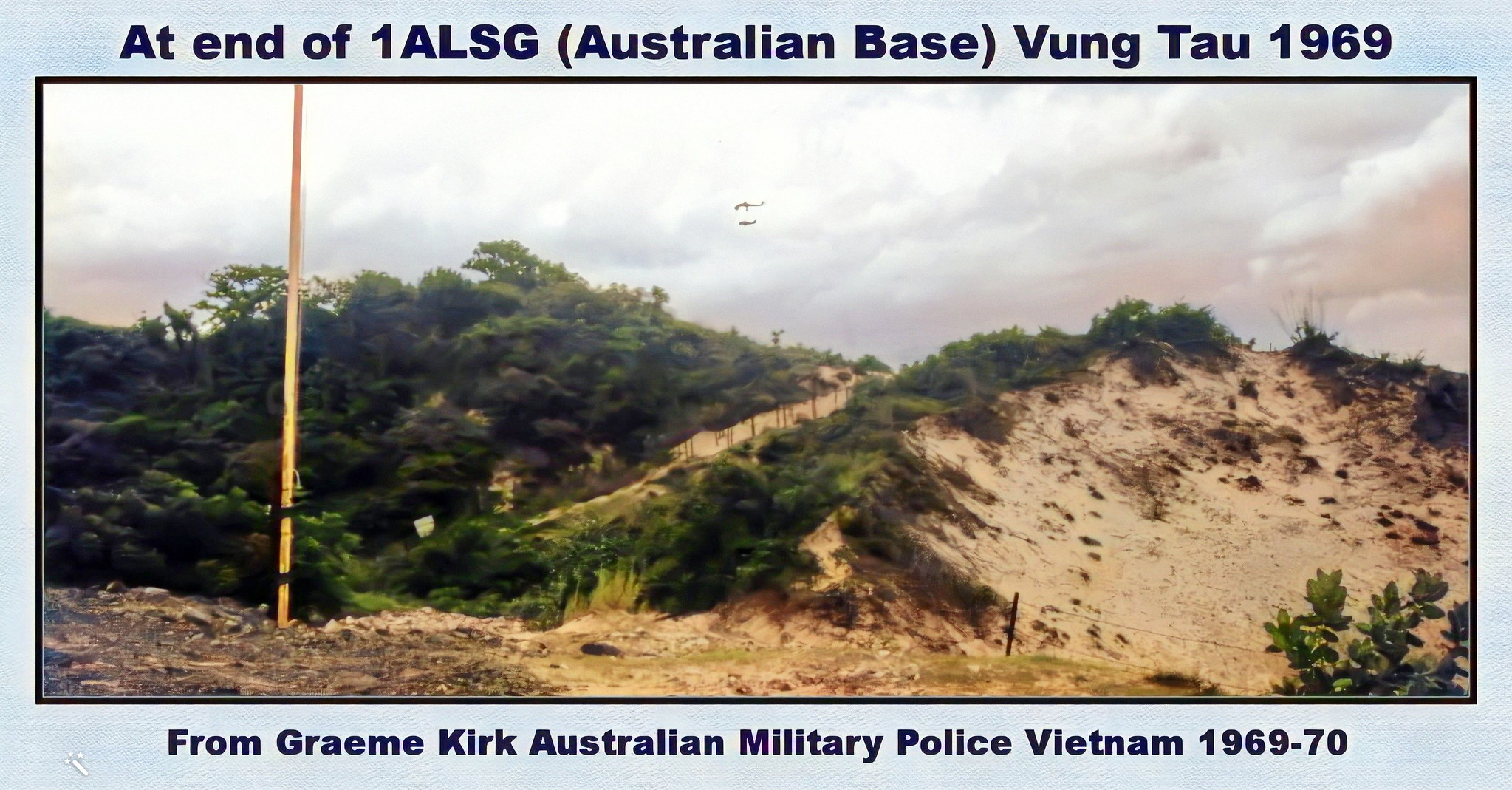The image captures a Vietnam War battlefield in vivid detail. Dominating the right side of the image is a towering sand dune or mound, contrasting sharply with the dense and impenetrable forest or jungle on the left. The sky above is filled with dynamic activity as helicopters fly against a backdrop of white and pink clouds. In the foreground, a solitary post or flagpole stands prominently, while sporadic stretches of metal wire fencing are visible throughout the frame, indicating fortifications. The top of the image bears the text: "At End of 1 ALSG, Australian Base, Vung Tau, 1969." Below, the caption reads: "From Graham Kirk, Australian Military Police, Vietnam, 1969-1970," providing both context and provenance for the photograph.